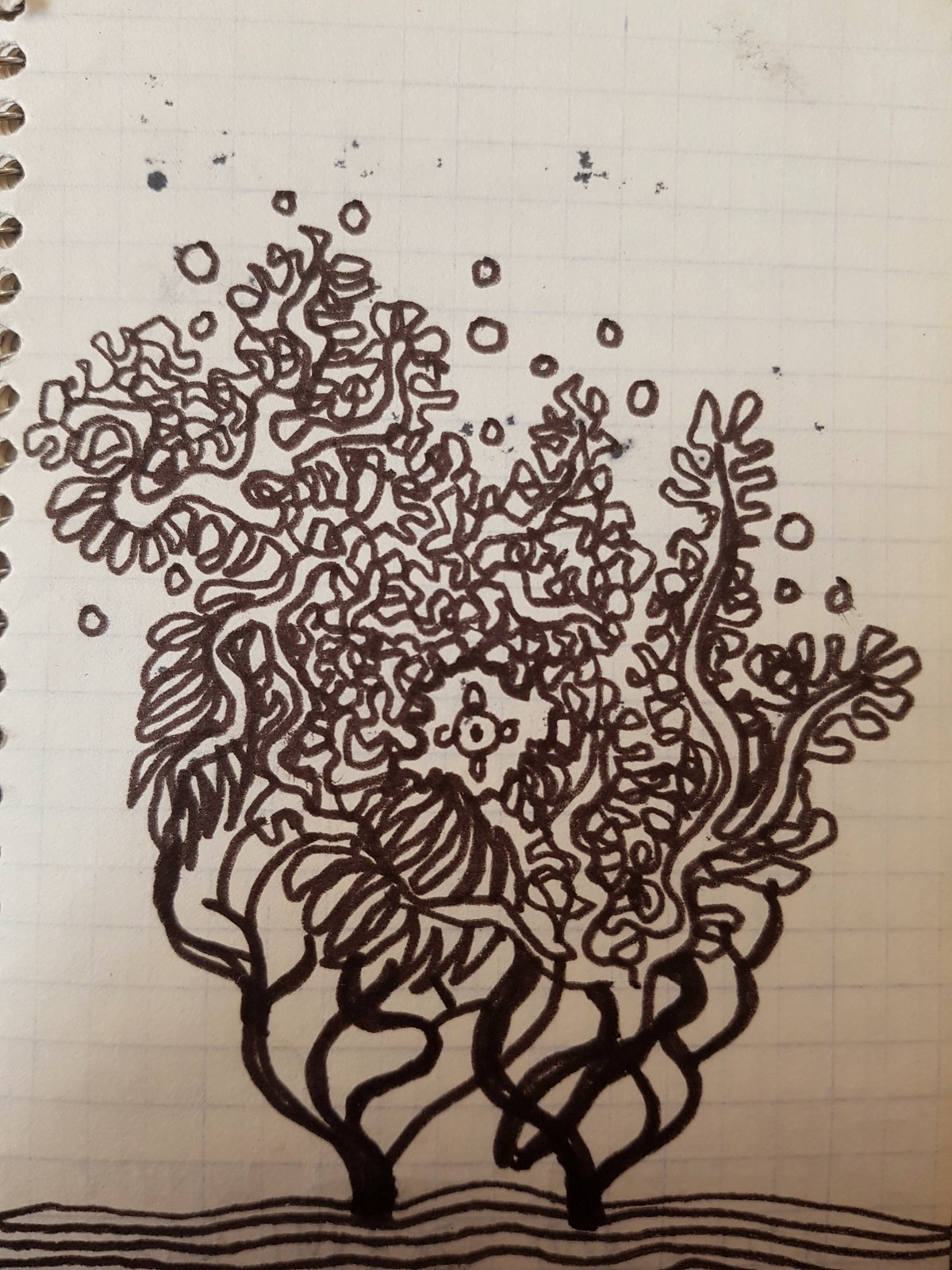This image features a predominantly brown-toned drawing on a sheet of graph paper. The artwork, occupying the majority of the sheet, depicts two stylized, bare-branched trees flanking the left and right sides of the paper. Their trunks rise from a curved, earth-like base at the bottom of the page. The branches extend upwards, intricate and leafless, filling the upper portion of the sheet with their sprawling, almost abstract forms.

The spaces between the branches are detailed with leaf-like shapes and an array of squiggly lines, creating a dense, textured canopy. Above the highest points of these tree-like forms, numerous small circles are scattered, giving the impression of scattered seeds or abstract fruits.

The left edge of the sheet reveals a portion of a ring binder, indicating the paper's origin from a spiral-bound notebook. Additionally, sporadic blotches from a marker or similar writing instrument adorn the top of the page, adding a casual, perhaps accidental artistic touch. The entire drawing is rendered in a rich, chocolate brown hue, lending it a cohesive and earthy aesthetic.